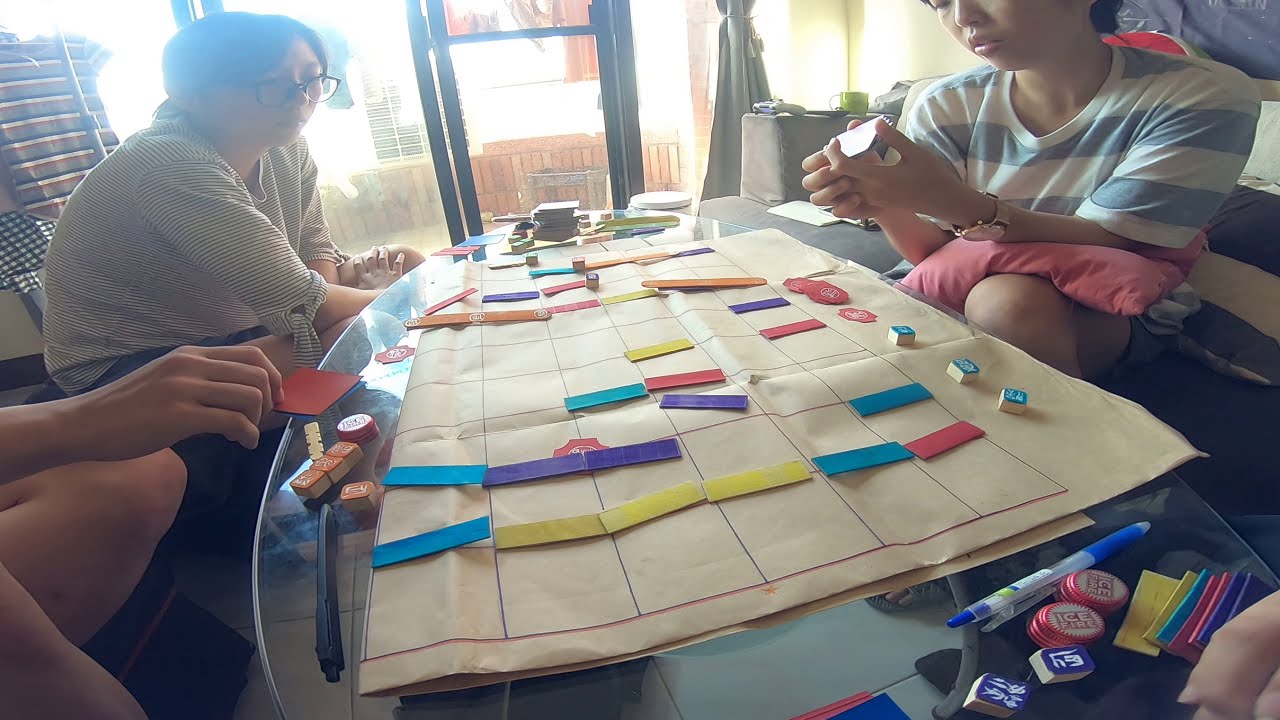This photograph captures a brightly lit indoor scene during daylight, featuring three individuals engaged in a board game at a rickety wooden table, which appears to be overlaid with a beige cloth grid. Two people are positioned on the left, and one on the right. The individual on the left is wearing a striped shirt and has a pillow on their knee, while the person on the right dons a white sweater. A partially visible arm and leg suggest another participant might be nearby. 

The game on the table involves various colored rectangular objects, aligned in the squares of the cloth grid, including yellow, purple, aqua, orange, and light orange pieces. Additionally, there are blue cube-shaped items with mysterious symbols, and piles of coins or poker chips scattered across the table. A pen is also present in the lower right corner of the table. 

Behind the players, the glass door opens to a bright patio, allowing ample natural light to flood the room, with more light entering from a window, enhancing the image's overall brightness. The scene conveys an atmosphere of concentration and engagement among the players.